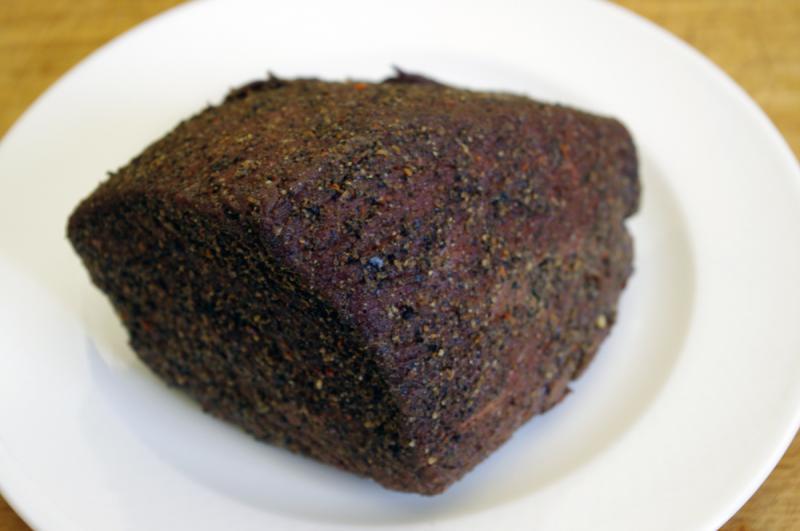The image is a detailed, close-up photograph of a heavily seasoned, well-cooked piece of meat resting on a stark white, circular plate. The plate features a slight depression in the middle and occupies most of the image. It is placed on a light brown, wood-grained table or butcher block surface. The meat itself is dark brown with a charred appearance, exhibiting rough, irregular edges and a dry surface, indicating it was likely transferred from another cooking vessel. Adorning the meat are numerous coarse seasonings, including black coarse pepper, and hints of blue, yellow, and white specks, suggesting an intricate seasoning blend. The meat shows some variability in color—shades of brown, pink, and gray—and is the focal point of the photograph, emphasizing its richly textured and seasoned exterior.